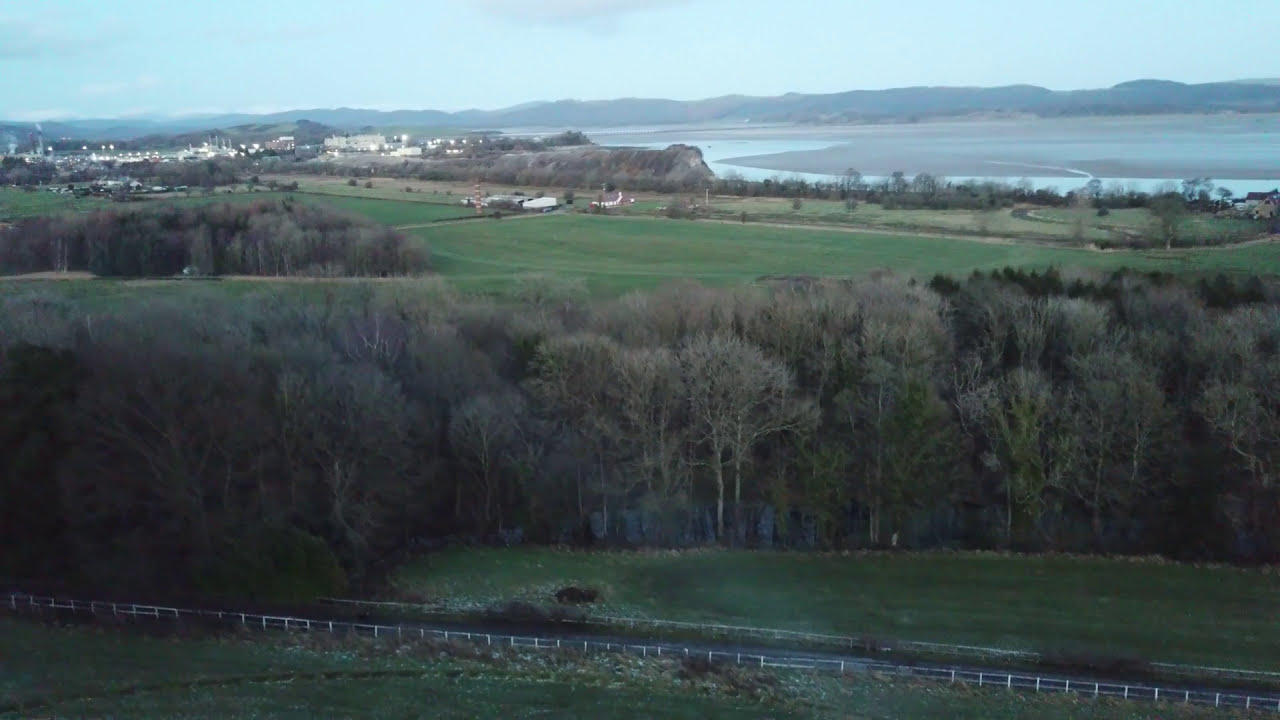This rectangular photograph captures a serene rural landscape transitioning from lush greenery to a distant town set against a backdrop of nature. In the foreground, a paved road traverses the image from the bottom right corner to the left edge, bordered by a green, grassy field. Adjacent to this field is a dense forest of tall, lush trees, with patches of both green and brown foliage. A long white plank fence, reminiscent of horse fencing, cuts across the front, adding a rustic element.

Beyond this initial stretch, expansive fields unfold, interspersed with groves of trees, particularly dense on the left. Continuing past the fields, a small cluster of farm buildings appears, suggesting a pastoral setting leading up to the town. The town itself, nestled into the background, features a variety of buildings with lights on, though their details are faint due to the distance.

Behind the town lies a large, tranquil body of water, possibly a lake, with its blue-gray surface reflecting the sky above. Bordering the water on the far side is a tree line, and beyond that, the serene vista is crowned by a distant mountain range stretching across the upper part of the photograph. The sky above is a light, hazy blue, adding a calm, peaceful ambiance to the scene.